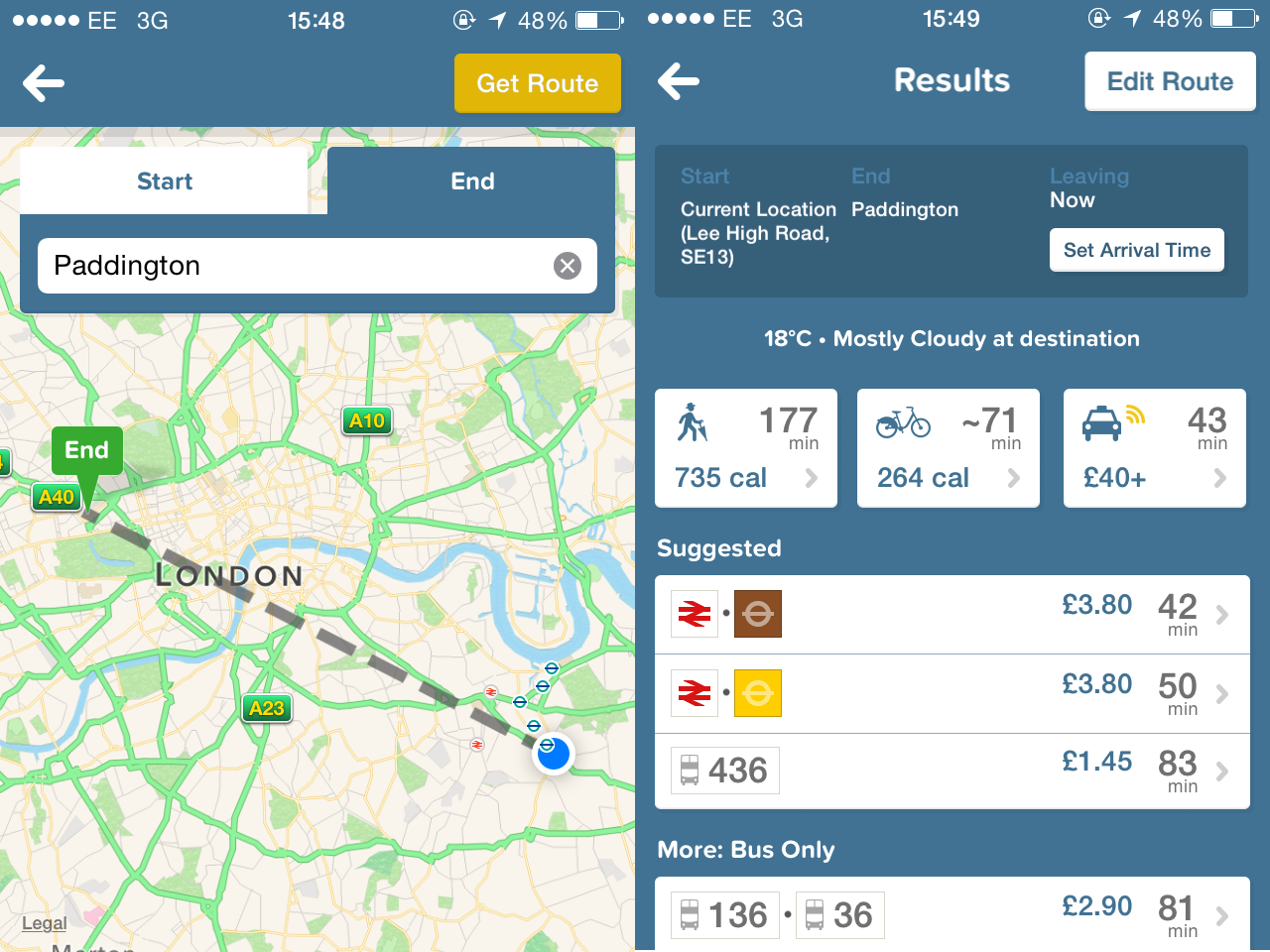This image displays a detailed navigation interface on a mobile device showing a map of London. The screenshot is split into two almost identical sections, side by side, with one showing the time as 15:48 and the other as 15:49. Both screenshots indicate a 3G network connection and a 48% battery life.

On the left side of the screen, there is an interactive map of London labeled with key highways such as the A23, A10, and A40. The map also prominently depicts the River Thames snaking through the city and various green lines representing different roads. A white arrow pointing left is located at the top, next to a yellow banner button labeled "Get Route." The user has input "Paddington" as the destination point. A blue circle marks the current location, with a grey dotted line indicating the route to the destination.

On the right-hand side, the detailed route information begins with the starting point, listed as "Lehigh Road SC13," and the destination, "Paddington." The current temperature at the destination is 18 degrees Celsius and mostly cloudy. The interface displays various travel times for walking, biking, and driving, alongside different public transportation options such as train and bus. It also includes the estimated pricing for each mode of transport.

This comprehensive display offers a clear visual and textual guide for navigating through London, complete with time, weather conditions, and transport options.